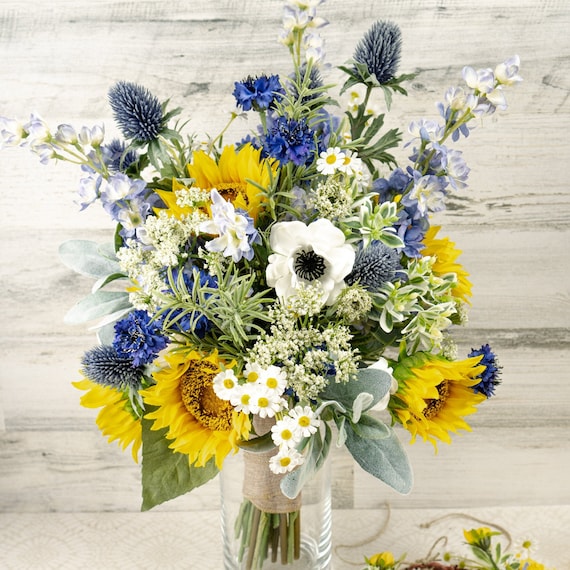The image captures a vibrant bouquet of flowers held in a clear glass cylinder vase. The stems, visible through the glass, are gathered together with a light brown ribbon. Dominating the bouquet are bright yellow sunflowers and a prominent white flower with a black center, likely a white poppy, positioned at the center. Additionally, the arrangement includes daffodils, light white-petaled flowers with yellow centers, and two types of smaller purple flowers—one in a poofy ball shape and the other with more ridged leaves. Blue flowers, along with blue and white blooms featuring yellow centers, add to the vivid mix, all interspersed with light green leaves and other greenery. Long stems with small purple and white flowers extend from the top, lending height to the arrangement. Positioned against a light-colored wooden wall, the bouquet sits on a white wooden surface, where some additional flowers are laid out beside the vase, enhancing the overall composition.